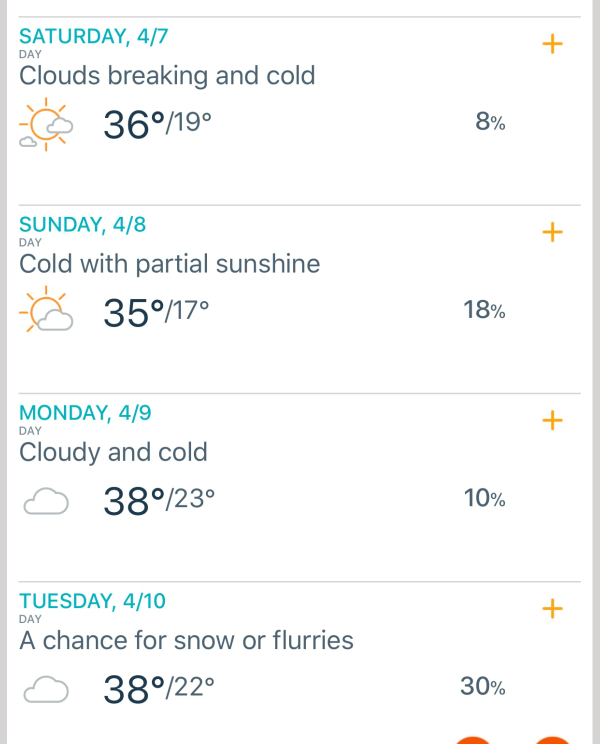This image captures a detailed weather forecast displayed on a cell phone screen. The screen is in a horizontal orientation, suggesting that more information may be accessible by scrolling up or down. The screen is bordered by two horizontal gray lines on either side, indicating the boundaries of the visible content. Thin gray lines separate different days, adding organizational clarity.

The forecast details each day with its name and date prominently displayed in teal. Below each date, a brief description of the weather appears in gray, followed by the temperature highs and lows in black. For example, the top entry reads "Saturday, 4/7." Beneath this, the description notes "Clouds breaking and cold" accompanied by a sun icon partially obscured by two clouds. The temperature is listed as 36°F / 19°F, where the lower value could either be in Celsius or the nighttime low. To the right, "8%" likely indicates a percent chance of precipitation.

Following Saturday, the subsequent days include:
- **Sunday, 4/8:** Forecasted to be 35°F and described as "Cold with partial sunshine."
- **Monday, 4/9:** Expected to be "Cloudy and cold."
- **Tuesday, 4/10:** Noted as having a "Chance for snow or flurries."

Given that this forecast discusses snow in April, it might pertain to a mountainous region or potentially somewhere in the Southern Hemisphere, such as parts of South America.